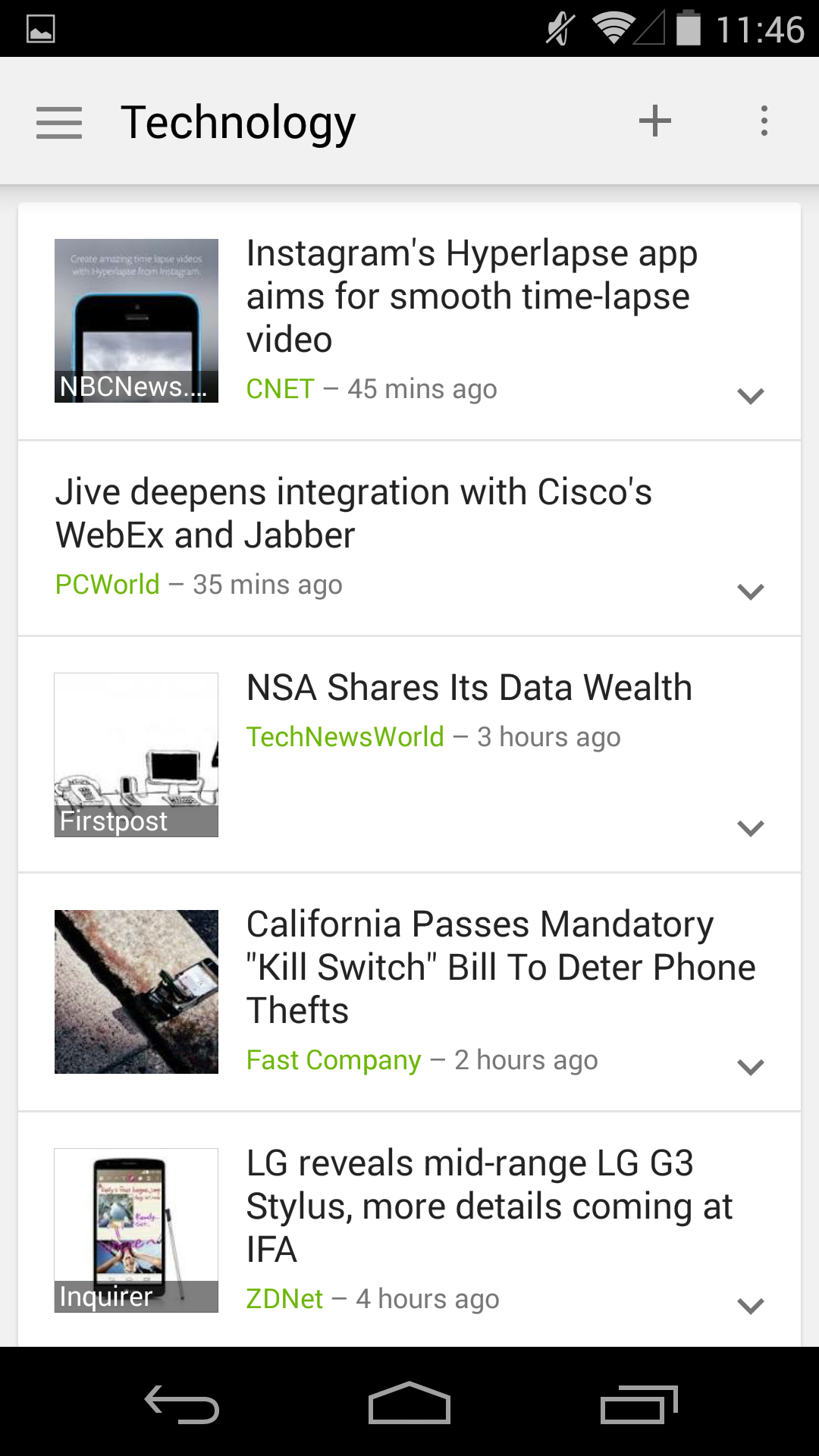A smartphone screenshot displaying a technology news page. The top border is black, featuring a picture icon on the left and a muted sound icon on the right. The Wi-Fi is active, and the battery is fully charged. The timestamp reads 11:46. Below, there is a hamburger menu on the left, followed by the word "Technology" in the center, and a plus sign with three vertical dots on the right.

The main content area includes several news items each in its own white box with a dropdown arrow. The first item shows the top edge of a smartphone screen with the NBC News logo, titled "Instagram's Hyperlapse app aims for smooth time-lapse video," noted as 45 minutes old. 

The second item, titled "Jive deepens integration with Cisco's WebEx and Jabber," from PC World, is marked as 35 minutes ago.

The third item includes a photograph of a desktop with an old hook-and-receiver phone, titled "NSA shares its data wealth," from Tech News World, 3 hours ago.

The fourth item displays a smartphone image and is titled "California passes mandatory 'kill switch' bill to deter phone thefts," by Fast Company, 2 hours ago. 

The fifth and final news item shows another smartphone, titled "LG reveals mid-range LG G3 Stylus, more details coming at IFA," from ZDNet, posted 4 hours ago.

At the bottom of the screen, there is a navigation menu with a backward return arrow, a home button, and an icon to lower the screen.